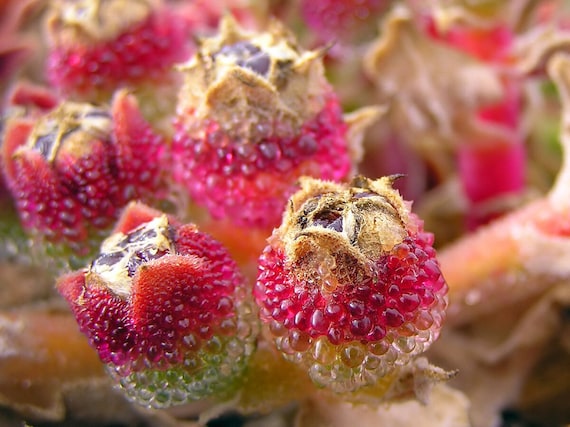This color photograph showcases a very close-up, detailed view of the buds of a common ice plant. The image, likely taken with a high-quality lens or magnification, highlights the intricate features of these pre-blooming plants. Each bud is characterized by a striking pinkish-reddish band near the top, transitioning into a more greenish-yellow hue towards the base. The buds also appear to have tiny, clear, gelatinous blobs on the outer sides, giving them a wet, dewy look. These blobs are reminiscent of small, fluid-filled sacs. The top of each bud appears to curl outwards, revealing small black bulb-like pieces within. In the forefront, two buds are sharply in focus, while the background fades into a blur, hinting at more buds. The plant's structure includes support sticks, and it all stands against a contrasting black background. An overhead, diffused light, suggestive of an overcast sky, illuminates the scene, adding to the soft yet vivid presentation of this unusual and captivating plant.